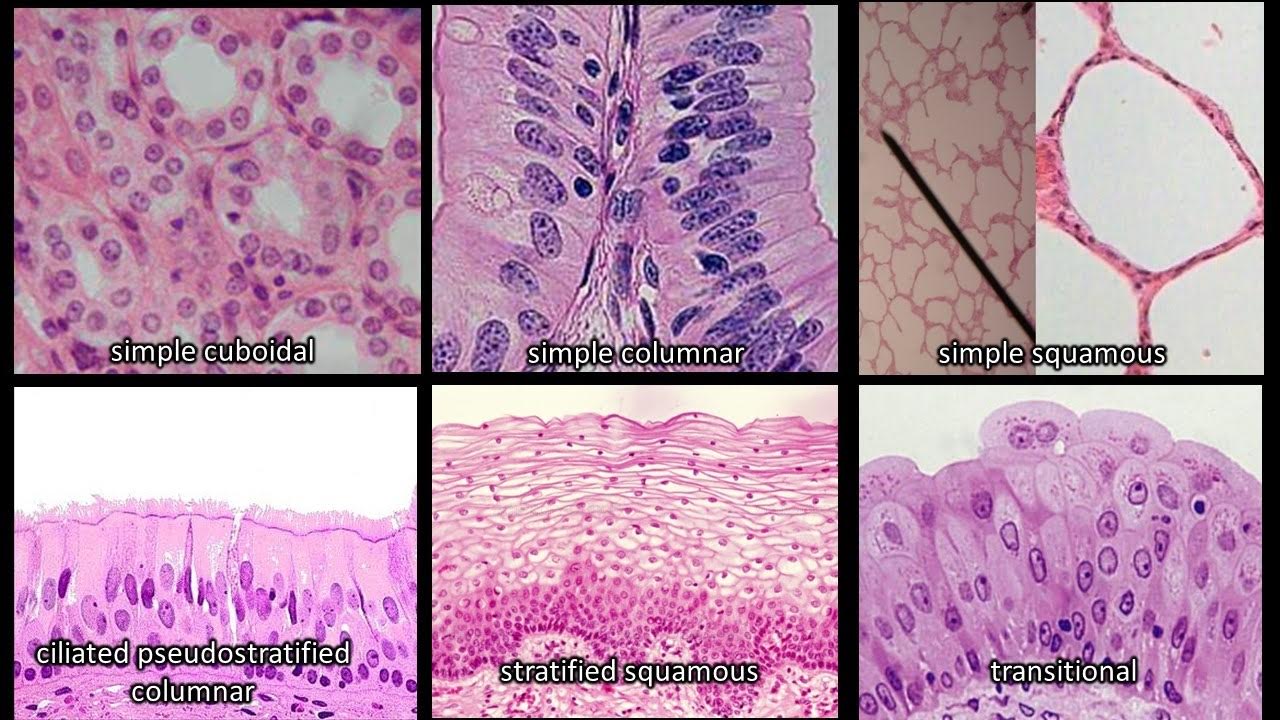This image is a collage of six highly magnified microscopic slides that showcase various tissue samples, all stained in shades of pink and purple to highlight cellular structures. The slides are organized in two rows of three. Starting from the top left, the first slide shows simple cuboidal epithelium characterized by pinkish circles with purple centers on a white background. Next to it, the second slide depicts simple columnar epithelium resembling a butterfly shape in light violet with darker purple spots containing tiny, dark purple circles. The third slide on the top row illustrates simple squamous epithelium, which appears similar to the inside of a cheek and is arranged in a circular formation.

On the bottom row, the first slide is labeled as ciliated pseudostratified columnar epithelium and appears purple, resembling grass with dark purple circular structures. The middle slide on the bottom is unlabeled and features a pink, stringy texture with numerous small dots. The final slide on the bottom right is also unlabeled; it has a purple hue and a structure reminiscent of a cactus, portrayed in tiny circular forms. All images have black borders, accentuating the vibrant colors and intricate details of the tissues.